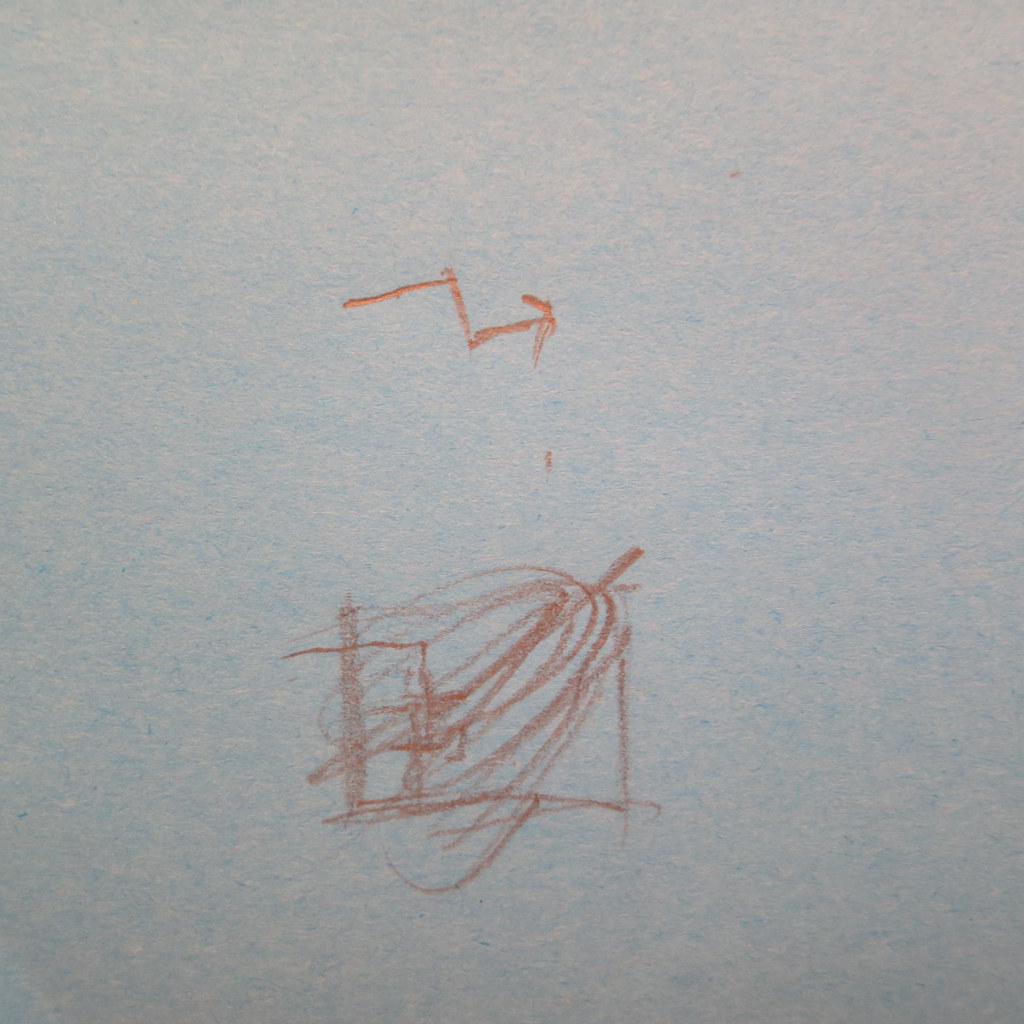A white sheet of paper serves as the backdrop for an abstract drawing composed of various scribbles. Dominating the top portion is a prominent orange mark, created with either a colored pencil or crayon, shaped roughly like an arrow pointing to the right. Just below the arrow, there is a series of pencil strokes that collectively form an irregular square. Inside this square, chaotic circular scribbles spill out, blurring the boundaries and creating a dynamic interplay between orderly shapes and free-form lines. The overall scene suggests a playful or experimental approach to drawing, where the constraints of conventional shapes are intentionally ignored.